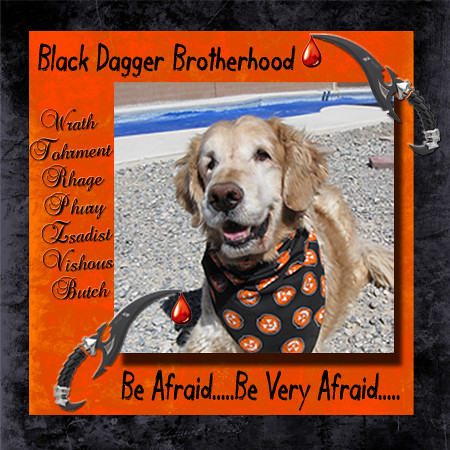The image is a square color photograph set against a vibrant orange background framed by a black border. The scene features a golden retriever standing on a sandy beach with a backdrop of blue water, looking up at the viewer with a friendly smile. The dog is adorned with a black neck kerchief decorated with orange jack-o'-lanterns, contributing to a playful, Halloween-themed aesthetic.

The top, left, and bottom of the orange background host black typography, featuring the headline in a stylish script: "Black Dogger Brotherhood" and "Black Dagger Brotherhood." Along the left side, various descriptive words are stacked vertically, while the bottom features the ominous phrase, "Be Afraid... Be Very Afraid..." in black text. Additionally, a blood-tipped curved steel knife is positioned at the top right, and another curved weapon is seen on the bottom left, blending photographic realism with illustrative and graphic design elements. The overall style is a striking combination of photographic realism, illustration, and graphic design, resulting in a humorous, condescending postcard-like advertisement that juxtaposes the harmless appearance of the golden retriever with a threatening theme.